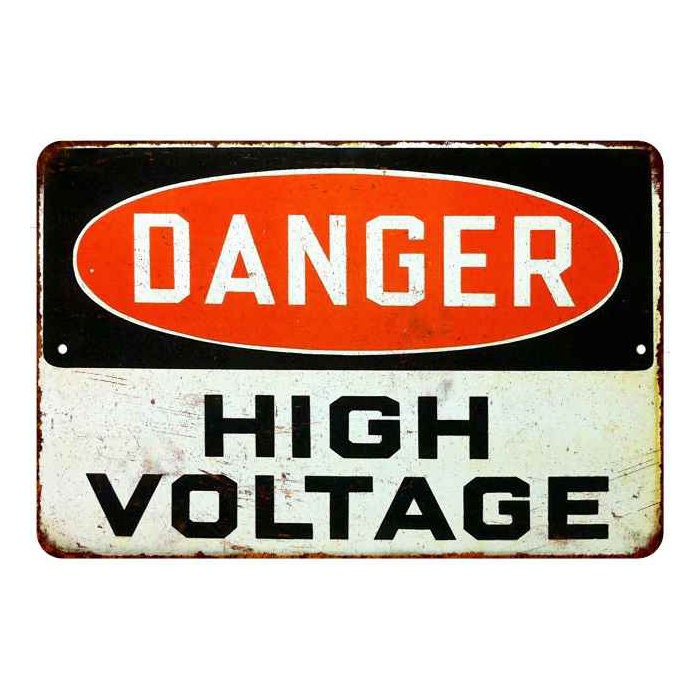This image depicts a weathered and rusted metal sign indicating "Danger, High Voltage." The sign is rectangular and shows significant signs of wear, suggesting long-term exposure to the elements. The top portion of the sign features a black background with a large, red oval shape that prominently displays the word "Danger" in bold, white letters. This section occupies roughly half the height of the sign. Below this, the background switches to white, where the words "High Voltage" are spelled out in large, black block letters. The entire sign is bordered by rust, particularly pronounced around the edges and corners, and the surface is marred by scratches and dirt. Additionally, there are two holes located on either side of the sign, designed for mounting it to a wall or fence. This sign appears functional yet distressed, hinting at its long-term service as a warning on a potentially hazardous structure or area.